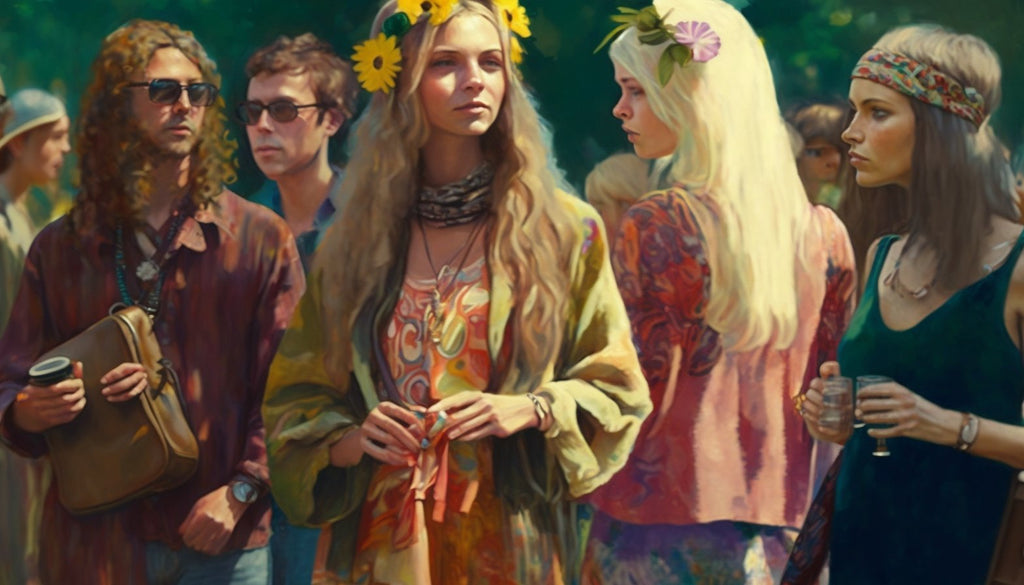The painting depicts a vibrant, festival-like gathering of hippies evocative of the Woodstock era, imbued with the classic hallmarks of 1960s counterculture. Central to the scene is a woman with long, wavy blonde hair, adorned with a crown of sunflowers. She wears a green and yellow long-sleeved blouse over a psychedelic-patterned sundress, composed of swirling orange, red, yellow, green, and blue hues. Her neck is draped with several necklaces, and a bracelet graces her left wrist as she gazes towards the right side of the image. To her right stands another woman, wearing a green tank top and a multicolored headband. This woman has light brown hair flowing just past her shoulders, and each of her hands holds a translucent glass with a stem. On the far left, a man with long curly hair and sunglasses holds a cup and a bag, with an unusual assortment of three random fingers emerging from the bag, suggesting the possibility of AI generation. Behind him, another man with short hair and sunglasses lingers. The overall backdrop includes blurry green foliage and indistinct figures, enhancing the dynamic and chaotic atmosphere typical of such gatherings.